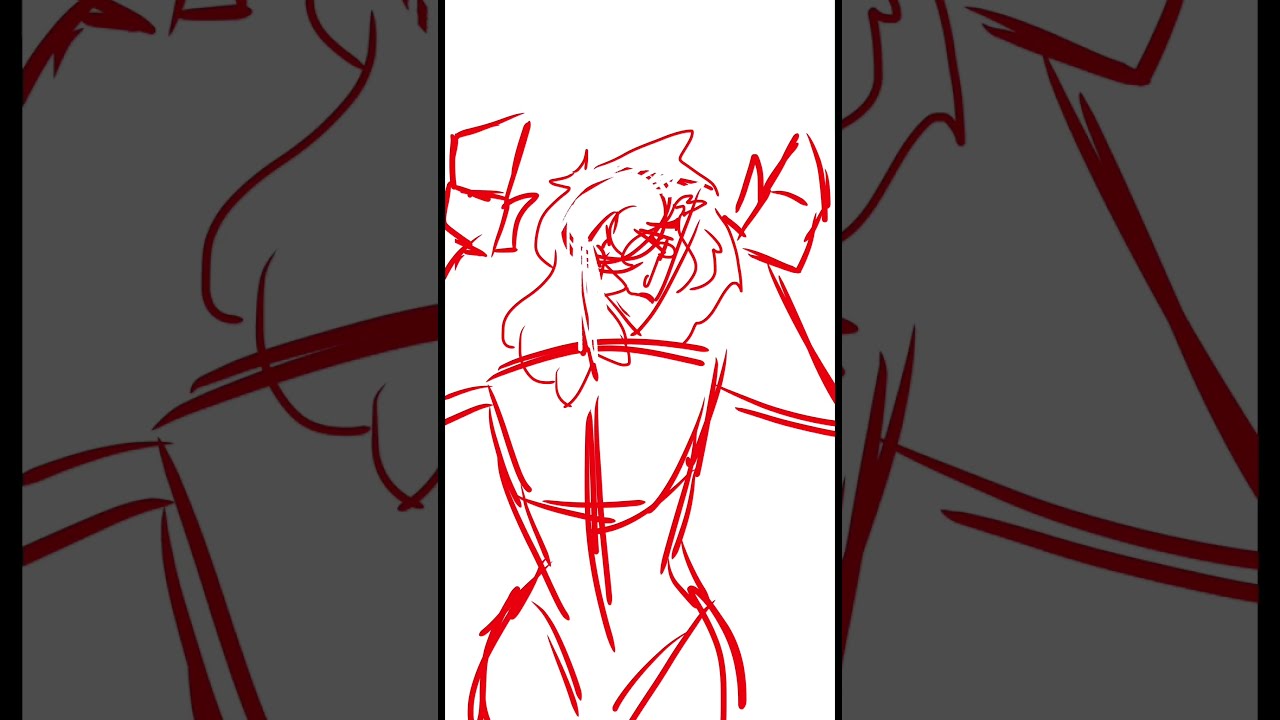The image presents an abstract digital sketch centered on a white background with semi-transparent, shaded sections on the left and right sides. The focal point is a dark red stencil-like drawing of what appears to be a mythical or fantastical creature. The creature bears a faint resemblance to a female figure, characterized by an hourglass shape, thin waist, and wide hips. Its head, positioned slightly above the center, resembles a dragon or has draconic features but is also interpreted as having long, wavy hair. The face has a discernible chin and a long smirk, with hair formed of erratic blobs in the front and spiky streaks at the back. The creature's body appears armored, featuring distinctive shoulder blade designs—pointy on the right and flat on the left ending in a corner peak. A cross symbol is prominently displayed on the torso. The incomplete sketch shows the arms raised, with stick-like, mitten-ended hands adding to its surreal appearance. The shaded side areas offer close-up segments of the red sketch but do not contribute additional clarity to the overall image. There is no text present in the artwork.